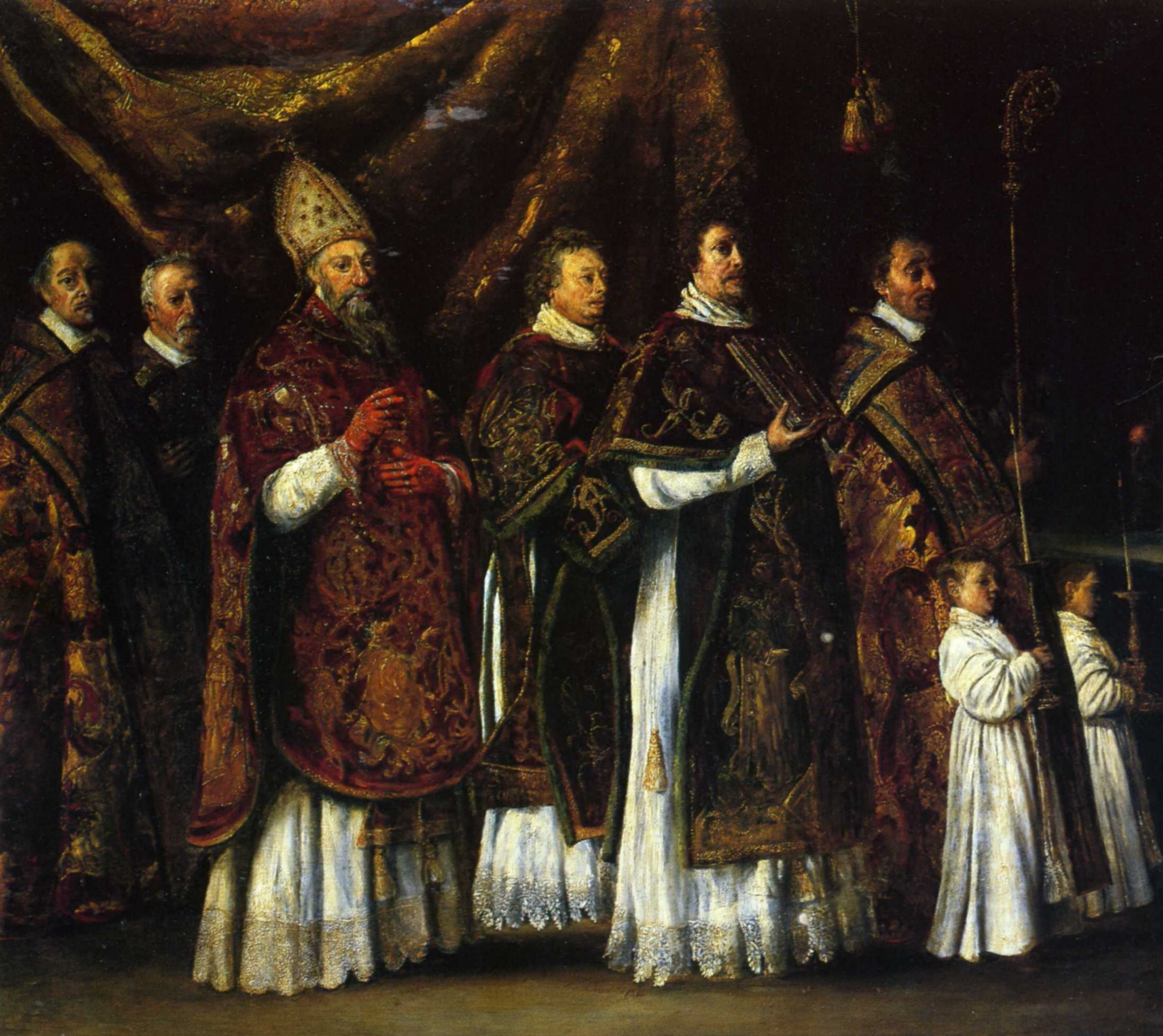The painting depicts a ceremonial scene with various religious figures, likely part of a Christian ritual. Dominated by warm gold and brown tones, the background consists of a decorative cloth draped over a wall, adding to the setting's solemnity. Centrally, an elderly figure, possibly a high-ranking church official like a Pope, stands out. He is adorned in a white tunic beneath a richly decorated red robe, accessorized with a headdress resembling a ceremonial helmet, and red gloves. This central figure holds a chain, amplifying his authoritative presence. 

Flanking the central figure are six men, dressed in ornate black and gold floral-patterned robes, indicative of their high status. They each feature grey or dark hair and beards, emphasizing their seniority within the religious hierarchy. To the right, two small children in white, long, and long-sleeved robes stand carrying religious symbols, perhaps sticks or tokens. Their positioning and attire suggest their role in the ceremony, underscoring the painting's focus on religious traditions and the continuity between the youth and the clergy.